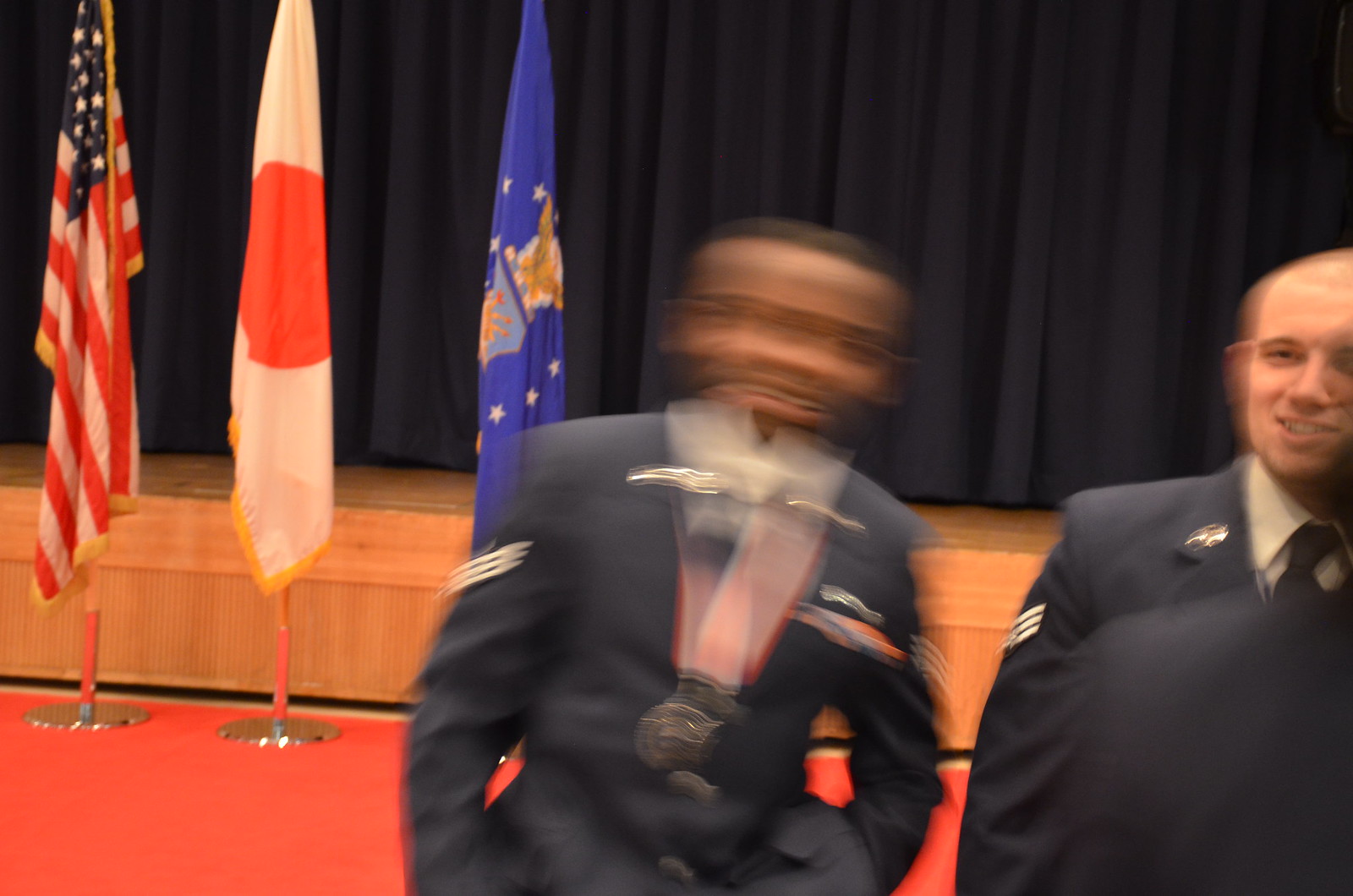The photograph captures a significant moment featuring two men standing on a stage. In the center of the image, there is an out-of-focus, dark-skinned man with very short hair, who appears blurred due to motion. He is dressed in a uniform resembling a military outfit, complete with a medal on a ribbon hanging around his neck. His arms are relaxed at his sides, with his hands tucked into his pants pockets.

To the right, another man stands more clearly in focus. He is white and also wears a dark blue uniform similar to the first man’s, accented with a blue tie and a white collar. Despite being slightly obstructed, more details are discernible about his appearance.

The backdrop of the scene is a stage made of natural-colored wood, veiled by a large, closed blue curtain. In front of the stage, three flags are prominently displayed on chrome bases with red poles, set against a red carpet. The flag on the left is that of the United States, the middle flag is likely Japan, identifiable by its white background and red circle, and the flag on the right is blue with an ornate coat of arms, although only partial sections of these flags are visible.